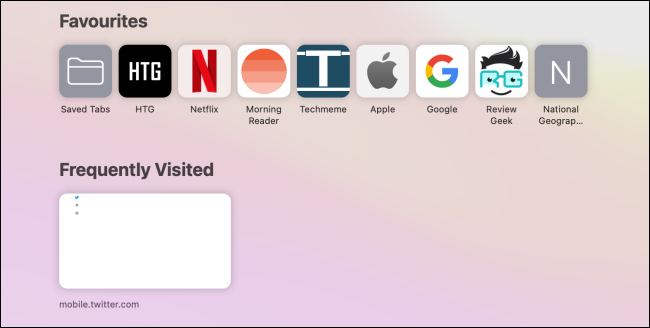The image is a wide, rectangular graphic with a light purple background, showcasing a neatly organized favorites section. In the upper left corner, the word "Favorites" is prominently displayed in bold black text. Below this heading, there are nine distinct icons, each accompanied by a label identifying it.

From left to right, the icons and their labels are as follows:

1. A gray square containing an image of a folder, labeled "Saved Tabs."
2. A black square with the white, capital letters "HTG," labeled "HTG."
3. A white square with a large red "N," labeled "Netflix."
4. A white square featuring a gradient circle transitioning from shades of red to lighter oranges and pale at the bottom, labeled "Morning Reader."
5. A black square with a white "T," labeled "Tech Meme."
6. A light gray square with an image of an apple with a bite taken out of it, labeled "Apple."
7. A white square with a multicolored "G," labeled "Google."
8. A white square with an illustration of a man's face wearing glasses, labeled "Review Geek."
9. A gray square with a black "N," labeled "National Geographic."

Below the collection of icons on the left side of the image, there is a white rectangle with no text inside. Beneath this rectangle, the text "mobile.twitter.com" is displayed. 

Overall, this detailed and organized graphic represents a user's favorite links or applications, each visually distinctive and clearly labeled for easy recognition.